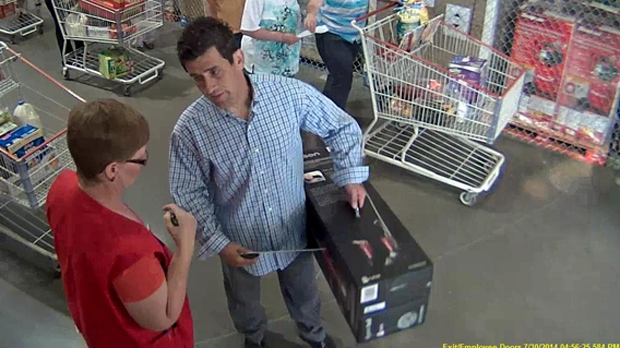In this bustling scene, the grey floor sets a neutral backdrop for the various activities unfolding within. At the center, a man with short brown hair stands out in his blue shirt adorned with black lines, which drapes over his grey trousers. He points with intent at a black box in his hand, his focus divided between the box and a nearby woman. The woman, donned in a white top with red and orange sleeves and stylish black-rimmed glasses, appears engaged in the interaction. Just behind this pair, a person maneuvers a grey shopping cart, loaded with items.

To their right, another duo is similarly occupied, each pushing grey shopping carts. These two are positioned near a fenced area that holds two red boxes resting on a crate. The person closest to the frame is dressed in black pants and a blue and white striped top, while their companion's long garment, featuring an intricate white and blue stencil design, is partially visible.

Adding to the layered visuals, another individual with a grey shopping cart can be seen further in the background, contributing to the scene's depth. At the very bottom left corner of the image, yellow lettered text appears, though it's partially cropped and unreadable, hinting at a possibly vibrant or informative signage just out of full view.